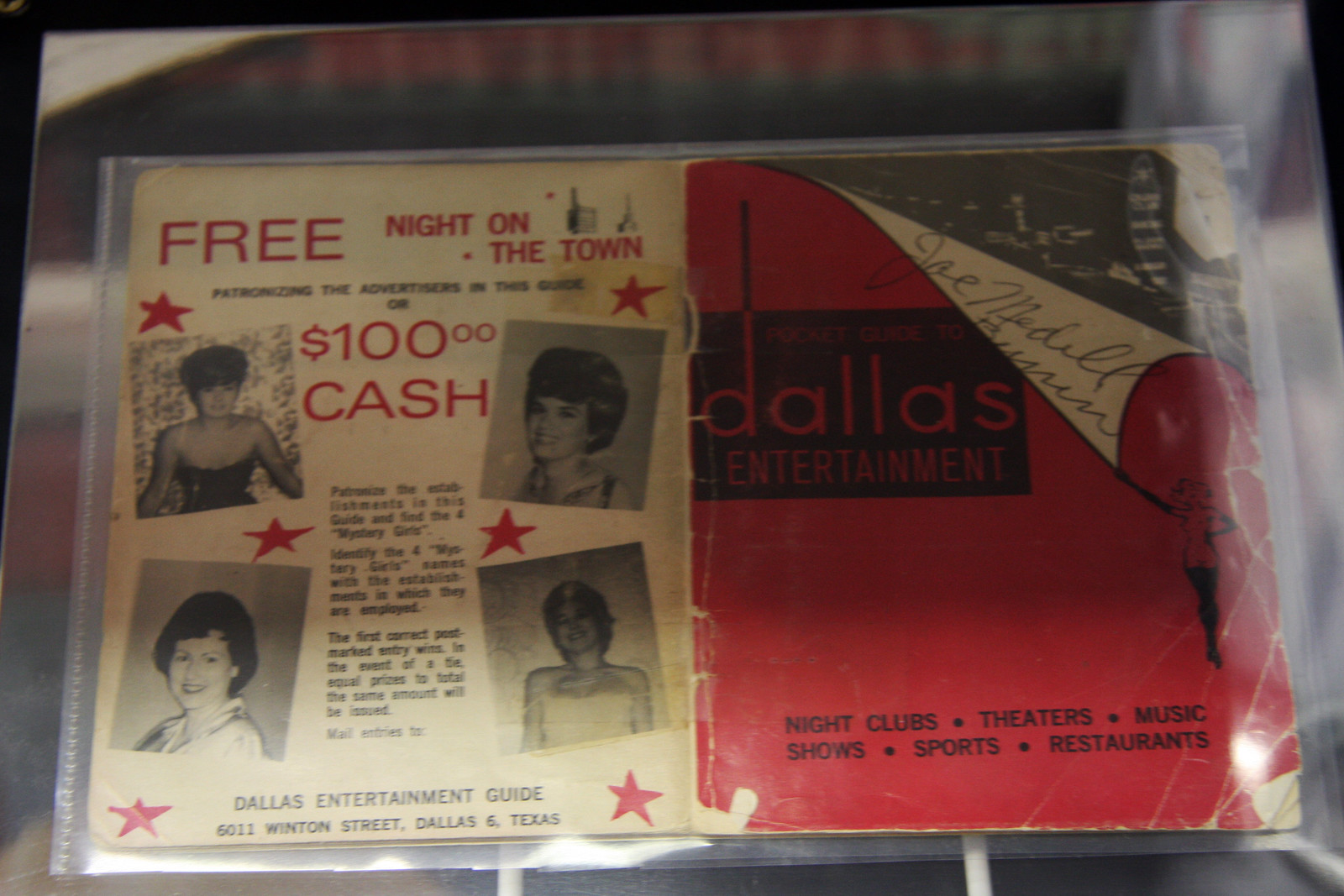This image captures an aged and stained magazine, likely from the 1940s or 1950s, encased in a protective plastic sleeve for preservation. The magazine is open, displaying the cover on the right side and the last page on the left. The right side, predominantly red, is titled "Dallas Entertainment" and offers information about nightclubs, theaters, music shows, sports, and restaurants. A striking illustration of a scantily clad woman in long black gloves and boots appears at the bottom right corner, seemingly pulling the page down. This side also features a handwritten signature that appears to be "Joe Middle."

The left side of the magazine, which is likely the last page, is primarily white with red and black text, and features four black-and-white photographs of young women. It advertises a "Free Night on the Town" or "$100 cash" for patronizing the advertisers listed in the guide. The text also includes an address for the "Dallas Entertainment Guide" located at 6011 Winton Street, Dallas 6, Texas.